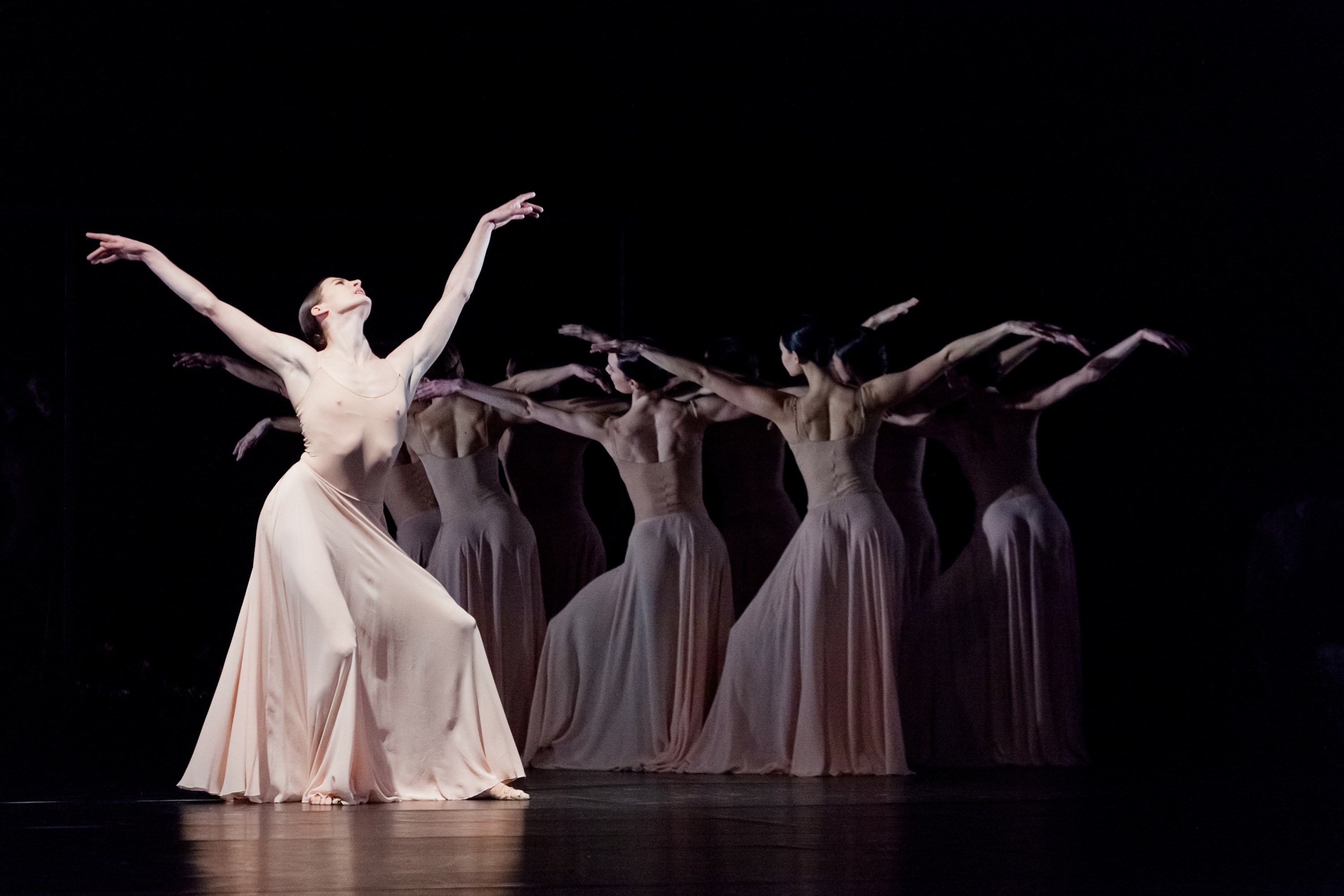The photograph captures a dramatic scene from a ballet or interpretive dance performance, set against a deep black background that accentuates the stage's dim lighting. Central to the composition is a woman in a light pink, sheer, ankle-length dress that clings to her body, revealing the contours of her legs, chest, and ribs. Her short-sleeved dress features a V-neckline. She is positioned slightly to the left and is illuminated by a spotlight, highlighting her pale complexion. She strikes a compelling pose, with her arms raised in a V shape and her head tilted back, her knees bent and pushed forward. Surrounding her in the darkness are approximately nine to ten other dancers, dressed similarly in long, flowing dresses. These background dancers echo her pose, some with arms extended to their sides, heads turned upwards or to the side, though they are less prominently lit, lending an air of mystery to the scene. The hardwood floor of the stage gleams faintly under the sparse lighting, enhancing the overall atmosphere of intensity and focus in the performance.